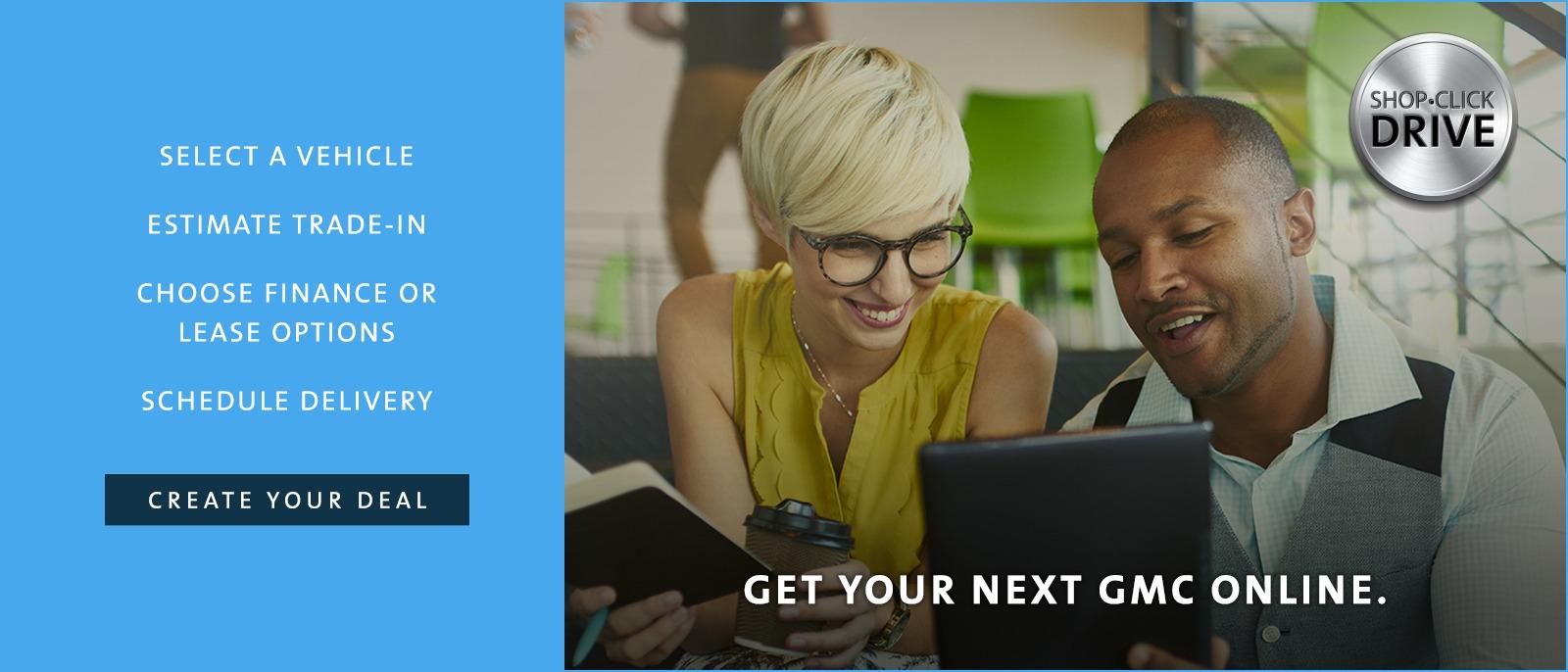The image is divided into two primary sections. On the left side, a blue background features a center-justified list in white capital letters, which reads: "SELECT A VEHICLE, ESTIMATED TRADE-IN, CHOOSE FINANCE OR LEASE OPTIONS, SCHEDULE DELIVERY." Below this list, a black rectangle contains white text that says, "CREATE YOUR DEAL."

On the right side of the image, a man and a woman are looking at a black tablet. The man, who has short black hair, a beard, and a mustache, is holding the tablet. The woman, with pinkish-brown skin, bleached white hair, and large brown glasses, is smiling at the screen. She wears a mustard yellow short-sleeved shirt, while the man is dressed in a shirt with a pattern of white, black, and gray.

In the top right corner of the image, a silver circle with black text reads, "SHOP CLICK DRIVE." Below this, in all capital white letters, it states, "GET YOUR NEXT GMC ONLINE." In the background, there is a green chair and another person standing. This person is wearing brown pants and a dark shirt, possibly black or navy blue. They are holding a book and a to-go coffee cup.